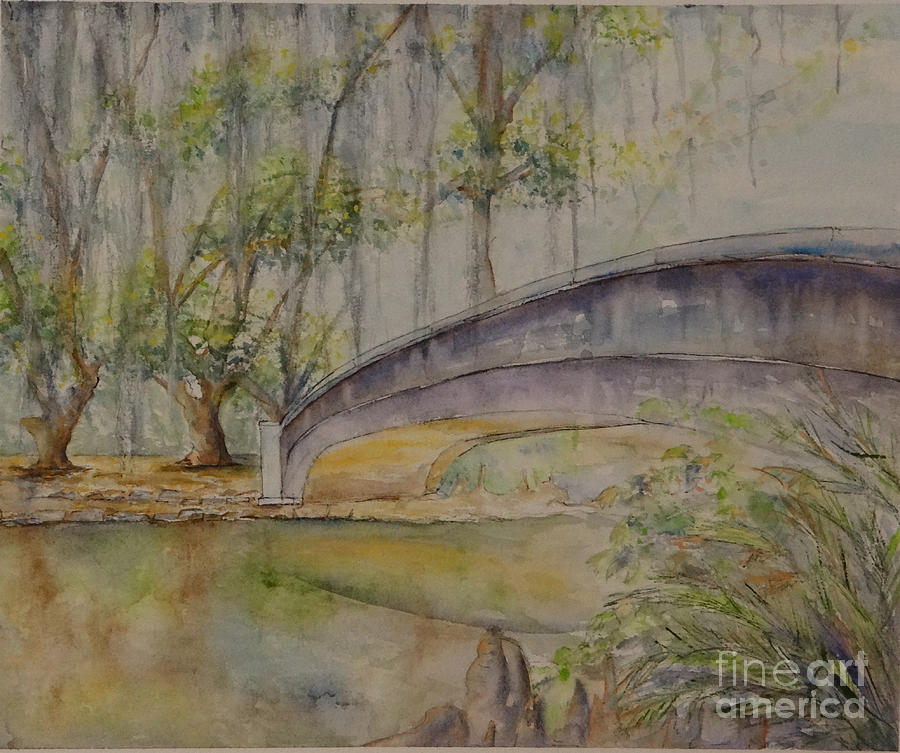A stunning Fine Art America piece, this image captures a serene garden or forest scene with a tranquil, gray-toned backdrop. At the center, a charming dirt path, rich with earthy browns, meanders up to a quaint, grayish bridge that spans a small, shimmering pond. Verdant green trees and plants envelop the scene, their long, delicate leaves and stems gracefully arching over. Splashes of green and blue hues from the foliage and water create a harmonious and peaceful setting, inviting viewers into this lush, natural oasis.